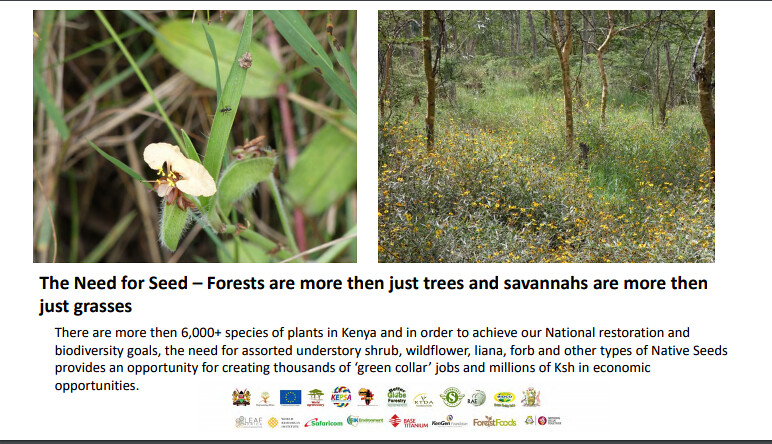The image is a wide rectangular screenshot, possibly from a website or a museum display, with a white background framed by thin black lines at the top and bottom. The focal point is two side-by-side images at the top. The left image is a close-up shot featuring a blade of grass, leaves, a couple of flowers, and several small bugs, including a prominent fly. The background consists of light brown and green string-like elements. The right image showcases a forested clearing with thin, widely spaced trees, tall grasses, and numerous yellow wildflowers. Below these images, the caption reads in bold black text: "The need for seed. Forests are more than just trees, and savannas are more than just grasses. There are more than 6,000 species of plants in Kenya. In order to achieve our national restoration and biodiversity goals, the need for assorted understory shrubs, wildflowers, lianas, forbs, and other types of native seeds provides an opportunity for creating thousands of green-collar jobs and millions of KSH and economic opportunities." The infographic emphasizes the critical role of diverse plant species in ecological restoration and economic development in Kenya.